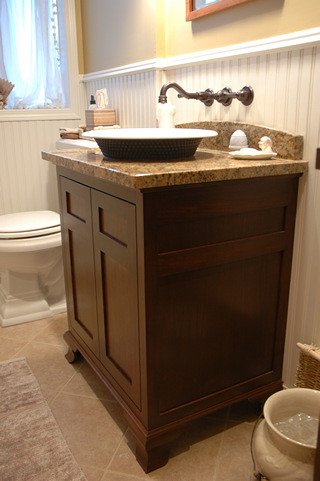This image captures an elegant segment of a well-appointed bathroom. The floor showcases tannish pink tiles with white grout, accented by a coordinating area rug in shades of pink and tan. Prominently placed in the bottom foreground is a large beige vase, contributing a touch of understated sophistication.

The right wall features a chic sink setup. A brown wood-toned cabinet supports a luxurious granite countertop, speckled with hues of tan, dark brown, and black. Sitting atop this countertop is a distinctive bowl sink, black on the exterior and white on the interior, with a dark bronze faucet and handle elegantly protruding from the wall above. The countertop also hosts a few decorative objects: a soap dish, a small carving of a human head, and an egg-shaped item that appears to be a room freshener.

The wall behind the sink is adorned with gray and tan striped wallpaper, bordered by a white trim. Above this trim, the wall transitions to a soft pink paint, enhancing the room's color palette. An art piece with a medium-toned wooden frame is partially visible at the upper part of the image. To the left of this artwork sits a window, allowing natural light to filter into the space.

Finally, the left side of the scene includes a toilet, topped with a box of tissues and a small bottle with a black rubber cap, providing a harmonious blend of practicality and style.